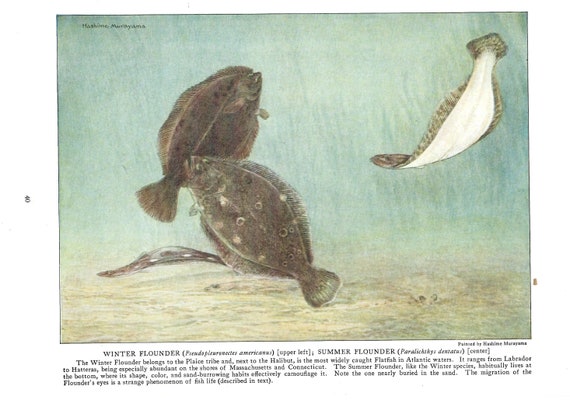The detailed, cleaned-up caption for the image would be:

"This is a detailed painting possibly executed in ink, watercolor, or oil, showcasing an underwater scene featuring four flatfish, likely flounders or flukes. The scene vividly portrays the sandy ocean bottom with yellow and brown streaks, and the surrounding murky, aqua-green water. Three of the fish are actively swimming: two centrally positioned, one facing left and the other right, and another hovering just above the ocean floor about to perch. The fourth fish, to the right, reveals its white underside. The flounders are characterized by dark greenish bodies adorned with brown spots, and subtle variations in their shading suggest differentiation between winter flounder and summer flounder, as indicated by partially legible text at the top and below of the artwork, although finer details are indiscernible. The overall shape of the artwork is slightly longer than it is tall."